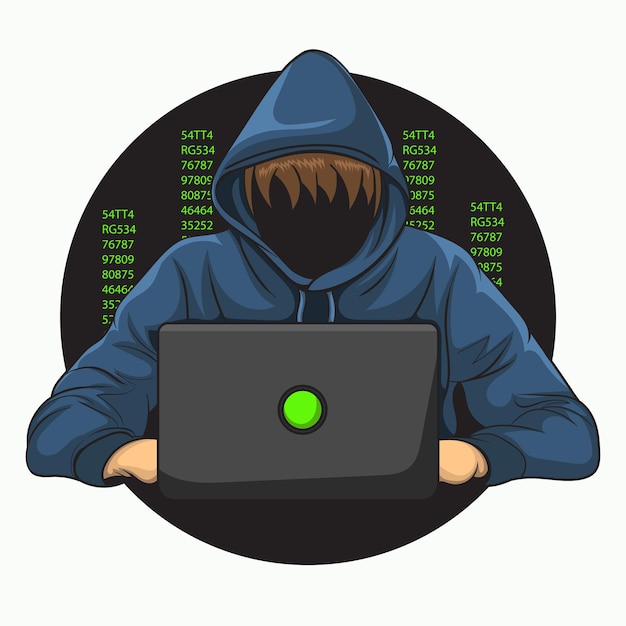In this digitally created or cartoon-style image, we see a character in a blue hoodie working intently on a gray laptop. The individual appears faceless, with jagged brown bangs descending over what should be the forehead. The head and much of the body are obscured by a large black circle superimposed over the figure. Within this black circle, a cascade of green numbers, resembling computer code, flows down the screen. These alphanumeric sequences include a mix of digits and letters, such as "5 4 T T 4 R T 5 3 4 7 6" located on the left side, and "3 5 2 5 2" centrally. Despite the lack of facial features, the person's Caucasian hands are visible, emerging from the hoodie sleeves to rest on the laptop keyboard. The stark white background contrasts sharply with the black circle and the vibrant blue of the hoodie, reinforcing the computer-focused activity, possibly related to hacking. The composition emphasizes the mystery and anonymity of the character, utilizing elements like the large black circle and cascading green code to enhance the sense of enigma and digital immersion.